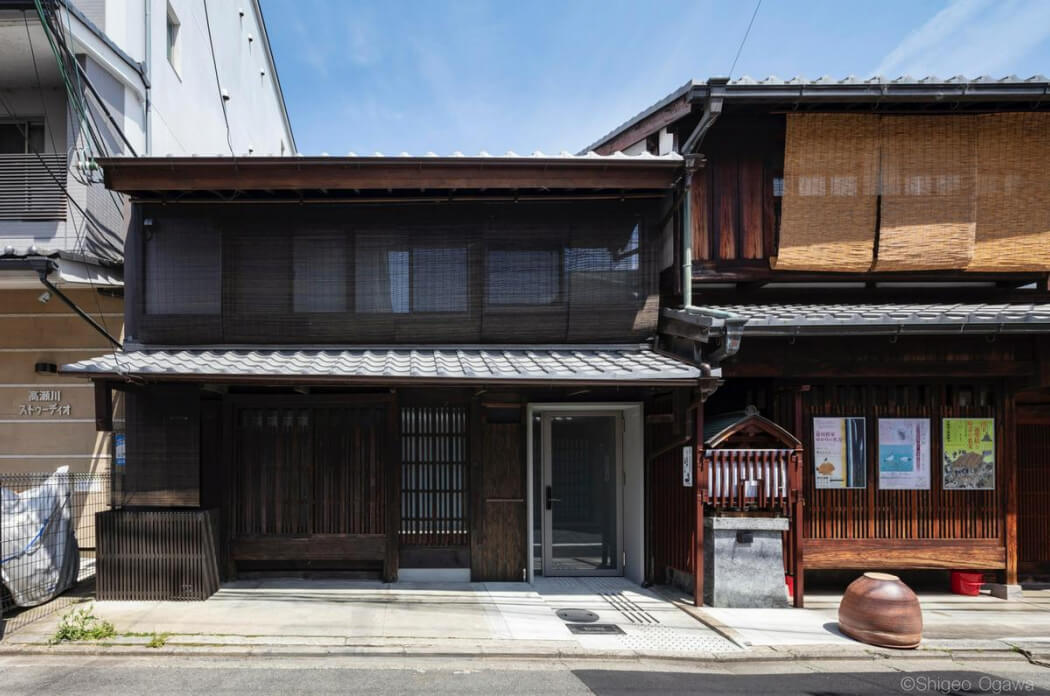The image captures a traditional Japanese neighborhood at street level, showcasing two adjacent buildings that contrast old and new architecture. The primary focus is on a two-story traditional Japanese house with a dark wood exterior and a flat, tiled roof. This house features a sheltered porch created by a slight terrace veranda roof. Its façade includes a glass door on the front and rolled-down mesh shades covering all the windows. Situated between two other buildings, the house on the right appears to be a slightly lighter wooden structure that could function as an inn, restaurant, or a similar commercial establishment; it also has mesh shades on the upper level and Japanese script on its front. Meanwhile, the building on the left is modern with Japanese lettering adorning its exterior. The photograph, taken during the day under a clear blue sky, shows the pavement and road extending across the foreground. A watermark at the bottom right credits the image to Shigeo Ogawa.